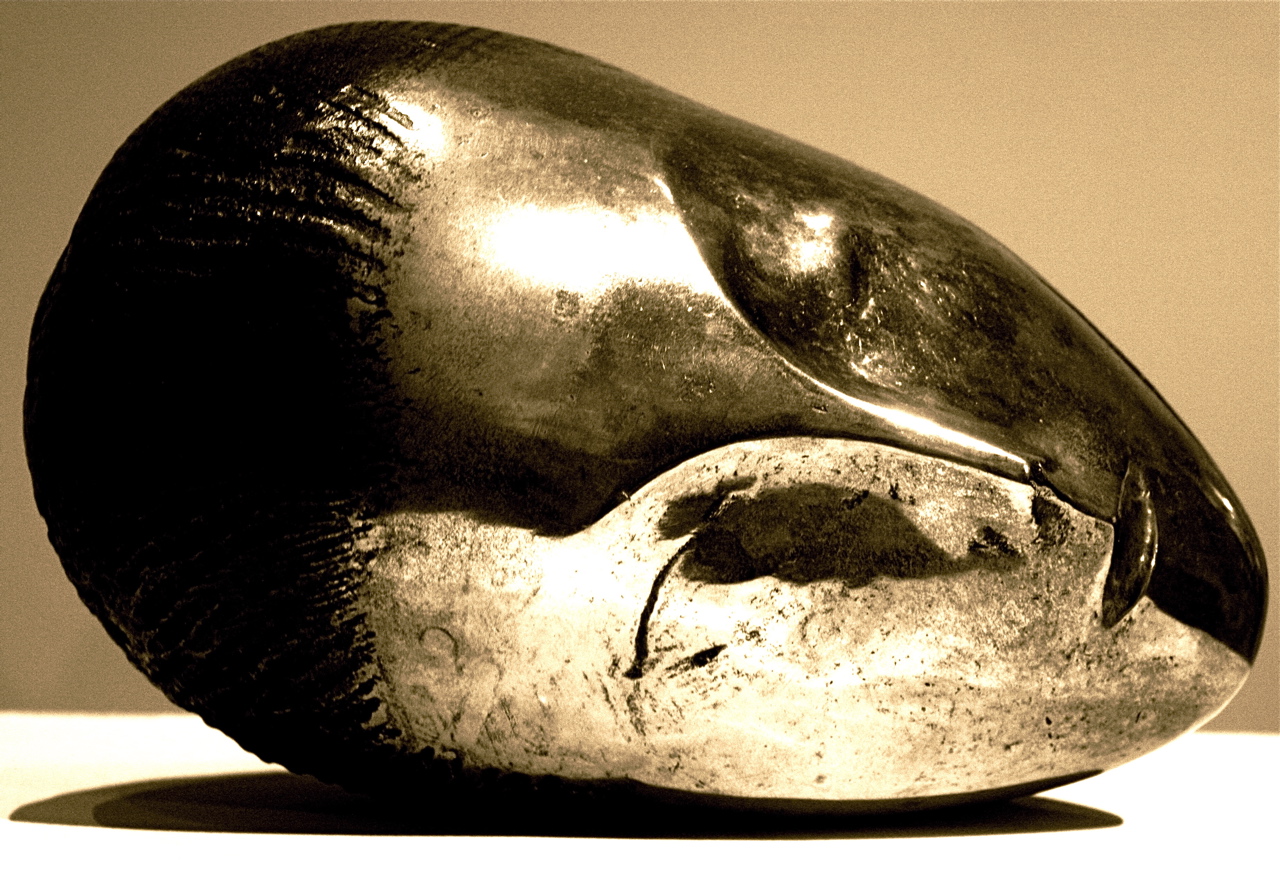The image depicts a striking, ancient-looking head sculpture or mask, oriented on its right side against a tan background with a brownish half-circle base. Crafted from a shiny metal, possibly brass, bronze, or a silver-like alloy, the mask has distinct features. The top of the head sports short black hair, and a noticeable indentation runs from the hairline down through the nose, dividing the face into two halves. The left side of the face shines more prominently, while the right side appears rougher. The mask features a very thin nose, indistinct eyes, and a small mouth with a black stripe extending from under it to the chin. The overall impression is that of an ancient artifact or possibly a masquerade mask, albeit with no openings for eyes, enhancing its enigmatic appearance.